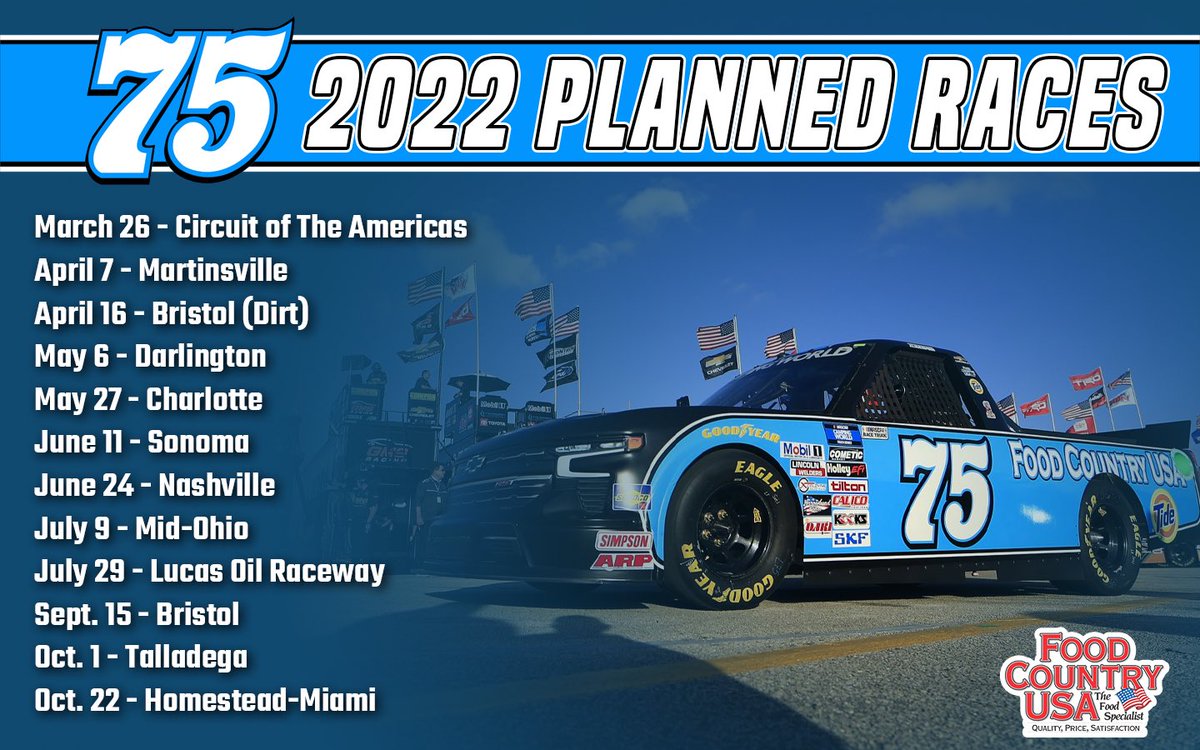The image is a horizontally rectangular, full-color print featuring a racing truck and accompanying text. The predominant theme color is blue. Across the top of the image, there is a blue banner with white text that reads "75-2022 Planned Races." 

Along the left side, the image lists the dates and locations of the races in white text. The dates and locations include: 
- March 25, Circuit of the Americas
- April 7, Martinsville
- April 16, Bristol
- May 6, Darlington
- May 27, Charlotte
- June 11, Sonoma
- June 25, Nashville
- July 9, Mid-Ohio
- July 29, Lucas Oil Raceway
- September 15, Bristol
- October 1, Talladega
- October 22, Homestead Miami

The center-right of the image prominently features a blue racing truck with the number 75 in white and the words "Food Country USA" next to it. The truck has a black top and black wheels with yellow text, reading "Eagle" and "Goodyear." The bottom right corner of the image has the text "Food Country USA" in red, all capitals, with smaller black text below that says "the food specialists" accompanied by an American flag. The truck's body is adorned with various advertisement stickers.